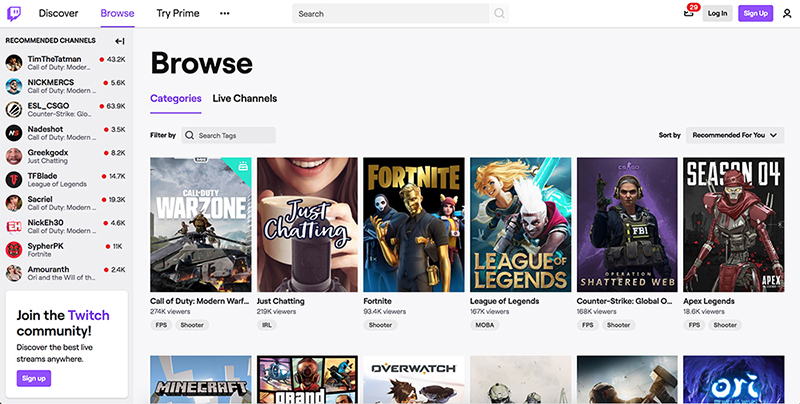This is a detailed screenshot of the Twitch interface, likely taken from a web browser. At the top left corner, the recognizable Twitch logo in purple is displayed prominently. Beside the logo, a menu bar features several options, starting with "Discover" in black. The "Browse" tab is highlighted in purple, indicating it is currently selected. To the right of these tabs, there is a "Try Prime" option and an ellipsis ("...") for more settings. 

Next to the ellipsis, there's a search bar for finding specific content, and a notifications bell icon with a red tab showing "29" notifications. Toward the top right, there are grey "Log In" and purple "Sign Up" buttons, followed by a profile icon depicted as a simple figure of a human upper body.

Beneath the menu bar, the main screen displays an array of games under the bold "Browse" heading, with the "Categories" section highlighted in purple. Other selectable options include "Live Channels." Several popular games are showcased here, such as "Call of Duty: Modern Warfare," "Call of Duty: Warzone," "Just Chatting," "Fortnite," "League of Legends," "Counter-Strike: Global Offensive," "Apex Legends Season 4," "Minecraft," "Grand Theft Auto," and "Overwatch." One partially visible game title looks like it could be "Ori something."

On the far left side of the screen, a list of recommended channels is shown, likely featuring notable streamers. The visible names include TimTheTatman, NickMercs, ESL_CSGO, Nadeshot, GreekGodX, TFBlade, Sacrial, NickEH30, CypherPK, and Amaranth. Below this list, a prompt invites viewers to "Join the Twitch Community."